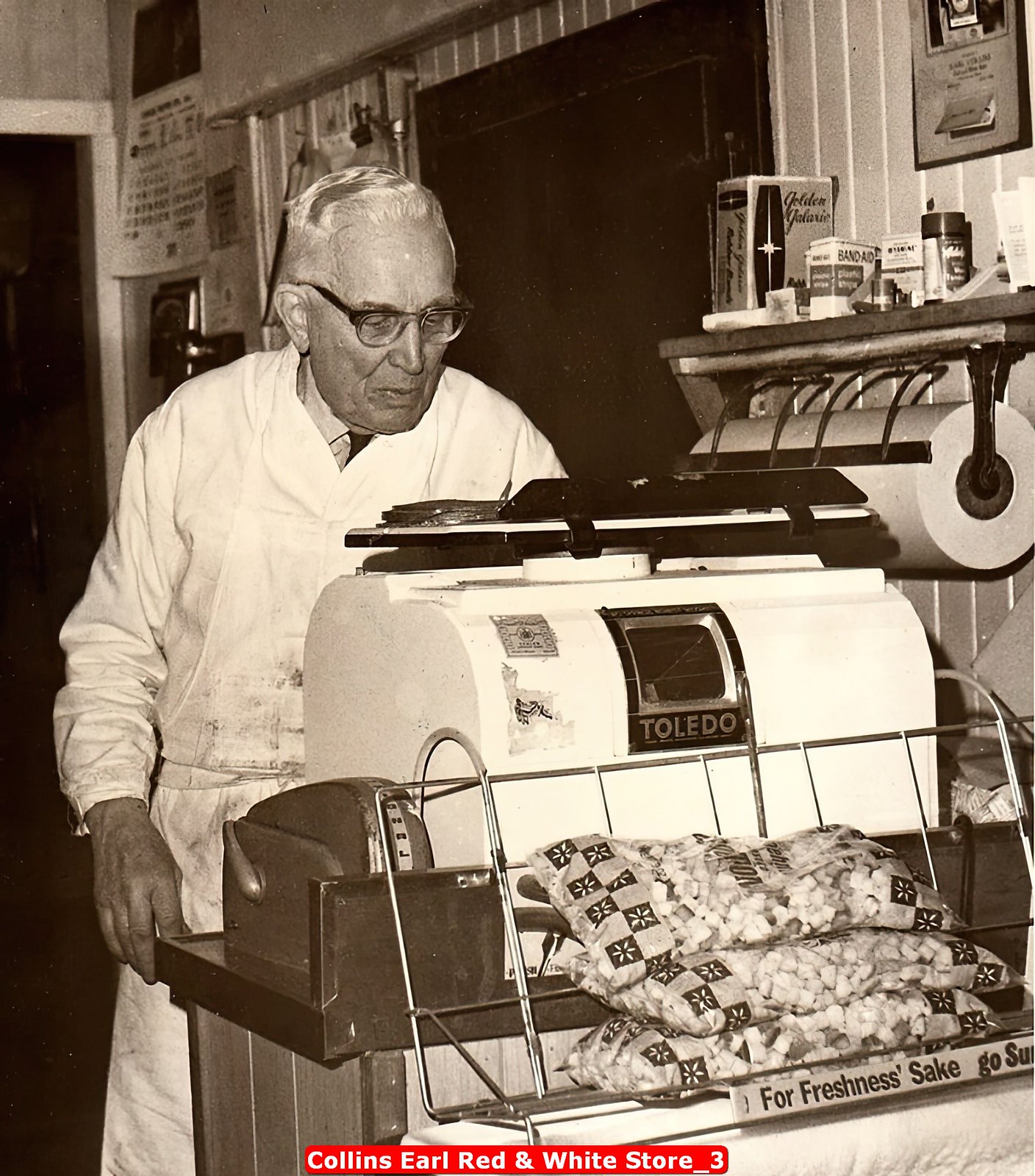This black and white photograph, possibly from the mid-20th century, captures an older man, likely a butcher, in a nostalgic store setting labeled "Collins Earl Red and White Store." The man, with white hair and eyeglasses, is dressed in a button-down collared shirt, a tie, and a white butcher's coat or apron. He stands by a machine marked "Toledo," which could be a meat slicer or a cash register. In front of this machine is a metal rack holding three bags of what appears to be food, possibly marshmallows or sugar, accompanied by a partially visible sign that reads, “for freshness sake, go” with the rest cut off.

To the right of the man is a large roll of white butcher paper on a shelf. Above this is another shelf displaying various items, including a metal tin of band-aids and a plastic jar of seasoning. The vintage ambiance is further enhanced by the presence of these period-specific details, evoking a sense of mid-20th-century commerce. The photograph exudes historical charm, capturing a slice of everyday life in a local store.